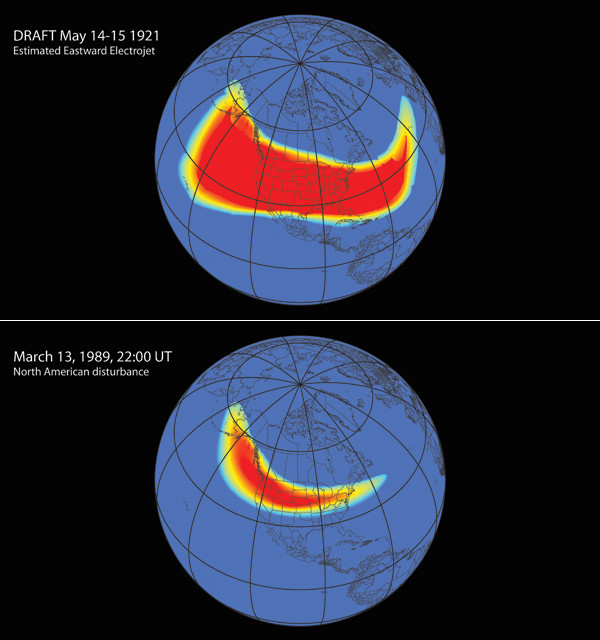The image displays two scientific diagrams of the Earth, both against a white background. Each globe is depicted in light blue with detailed black outlines of states, countries, and landmasses, accompanied by lines of longitude and latitude. The top image, marked with the text "Draft May 14-15, 1921, the estimated eastward electric jet" in white on a black background, illustrates a large red amorphous blob with yellow and blue outer edges, covering most of the United States and extending into the surrounding oceans. The bottom image is labeled "March 13, 1989, 22 UT, North American disturbance" and shows a similar but significantly smaller red region, predominantly over the northern and midwestern United States and stretching slightly toward Alaska. Both diagrams highlight red areas indicating disturbances or significant scientific observations over North America during the designated time periods.